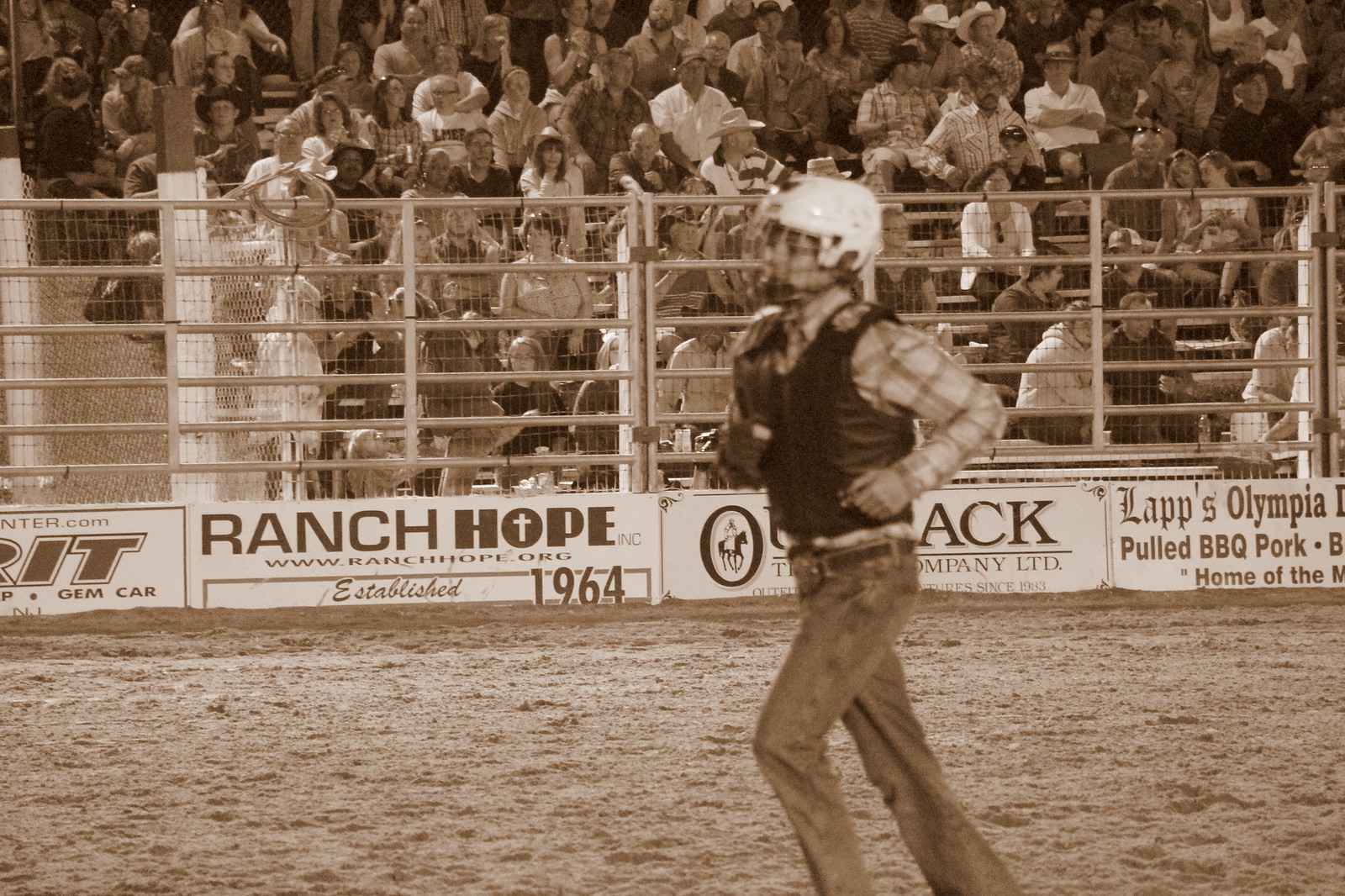This black and white photograph depicts a rodeo scene, likely from the 1960s, as suggested by an advertisement indicating "Established in 1964" for Ranch Hope. The central figure is a rodeo participant running across the dirt infield, dressed in typical rodeo attire including a white helmet with a face cage, a protective vest, a shirt, jeans, and a belt with a large buckle. The participant appears to be moving to the left side of the frame. The background showcases a large, engaged crowd with many spectators standing, cheering, and seated in the stadium benches. The stadium is secured with a metal, chain-link fence with bottom panels, possibly for added safety to prevent any potential incidents involving runaway bulls or horses. Advertisements are visible at the bottom of the fence, including promotions for "Ranch Hope" and "pulled barbecue pork," suggesting some connection to contemporary sponsorship or events.